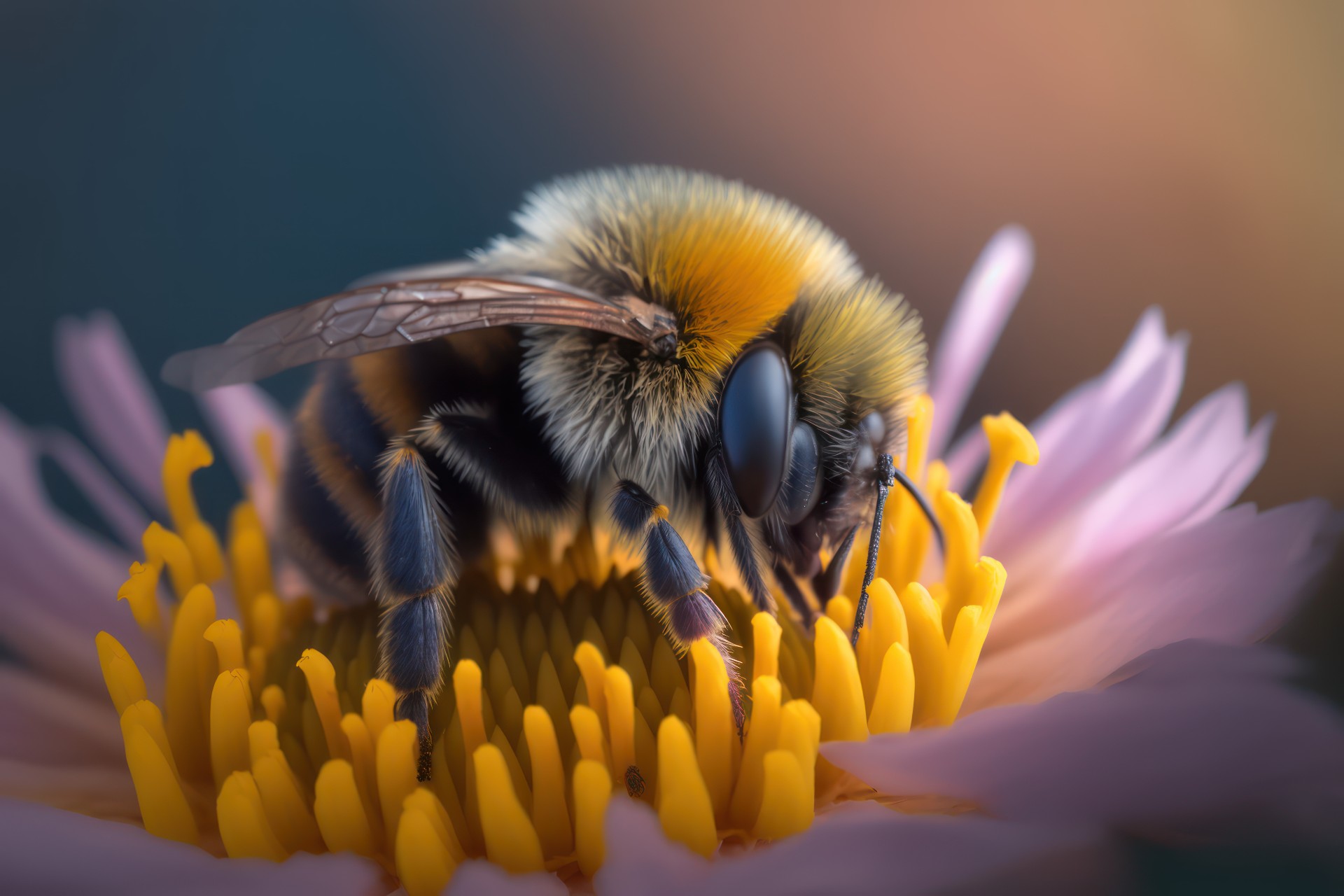In this captivating close-up image, we see a detailed shot of a bumblebee immersed in gathering nectar from a fully open pink daisy. The bee, with its slightly orange and yellow furry body, black legs, and almost translucent wings, is diligently collecting pollen from the bright yellow central part of the flower, with its head deeply dipped into the bloom. The daisy’s petals are pale pink, surrounding a striking yellow center where the bee is focused. The background is beautifully blurred, with hues of blue in the top left, pale orange in the top right, and purples fading into pinks at the bottom, accentuating the vibrant colors of the flower and the bee. The bee, facing towards the right, also has noteworthy features like its big blue eyes and fluffy, white-and-gold back. The intricate details, from the texture of the bee’s “fur” to its delicate, light copper wings, are sharply captured, showcasing the fascinating interaction between the bee and the flower.